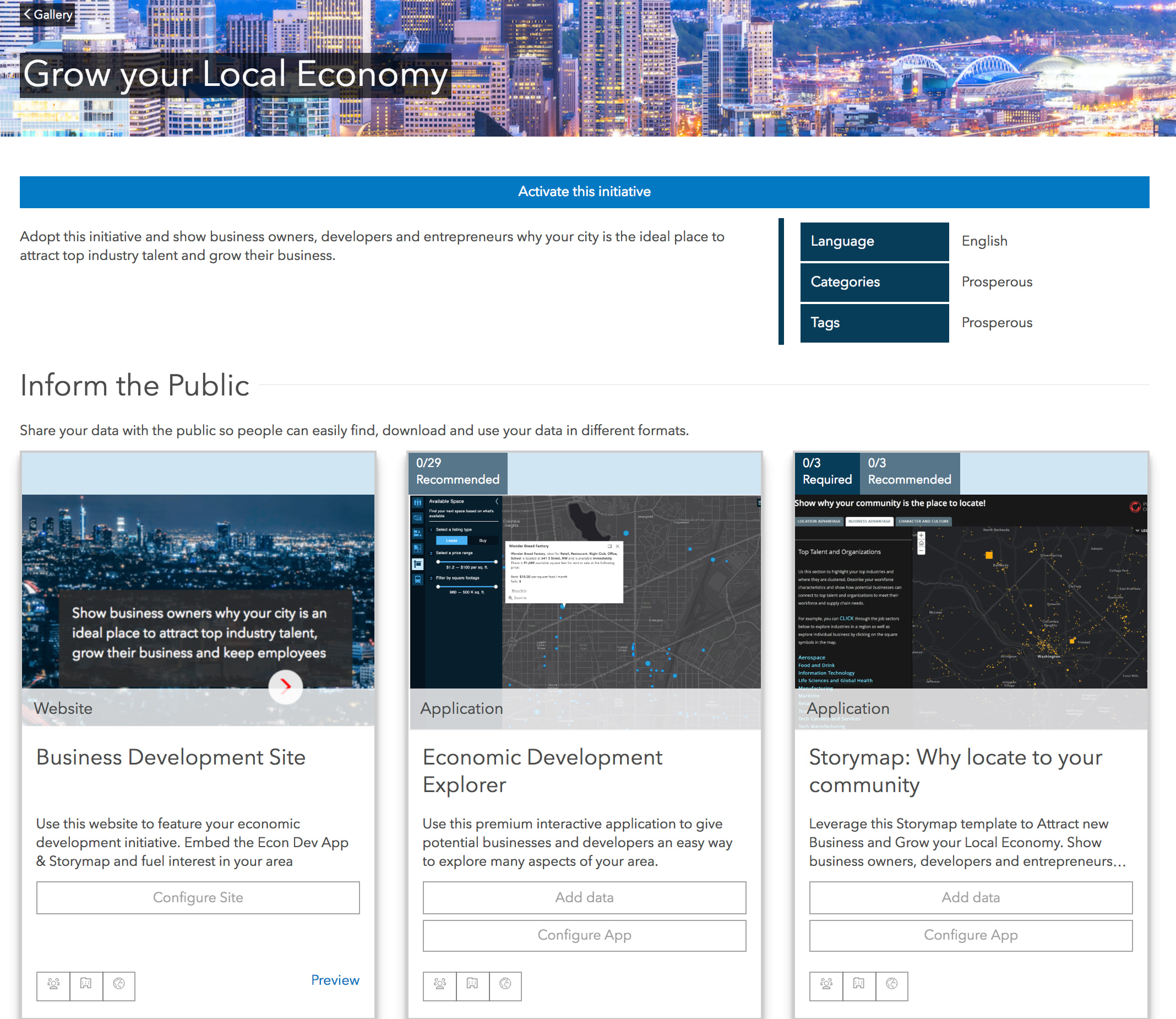The image is a screenshot of a website geared towards promoting local economic development. Dominating the header is a vibrant picture of a night sky filled with high-rise buildings, bridges, and an array of twinkling city lights over a translucent black field. On the left side, the text “Grow Your Local Economy” is prominently displayed. There’s also an option to return to a gallery.

Below the header image is a large blue bar with the call-to-action message: “Activate Your Initiative. Adopt this initiative to show business owners, developers, and entrepreneurs why your city is an ideal place to attract top industry talent and grow their business.”

To the right, there are settings for language, currently set to English, and options categorized under “Prosperous” with corresponding tags.

Underneath this section is another header reading “Inform The Public,” followed by three vertically aligned panels designed for smartphone viewing. These panels enable sharing data with the public in various formats. Each panel features images—a night shot of the city, a Google Map view, and a darker Google Map view.

The panels are tagged with labels like “Website,” “Application,” “Business Development Site,” “Economic Development Explorer,” “Story Map,” and “Why Locate to Your Community.” Each panel includes explanatory text and buttons for configuring the site. The middle and right panels further include options to “Add Data” or “Configure the App.”

At the lower part of each panel, there are three small icon buttons, though their specific functions are unclear from the image.